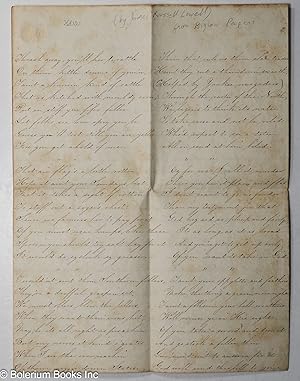The image is a photograph of an old handwritten letter, possibly several decades to over a century old. The entire page is filled with cursive writing in black ink, with a distinctive slanted style where the letters lean forward. The paper itself is primarily a dull white, showing significant signs of aging with dark brown discolorations, especially around the edges. There are visible watermarks of "Blenheim Books Inc." at the bottom left corner, and the page appears to have minor water damage and some folded areas. Despite its age, the letter is in good physical condition with intact corners and no tears, although the handwriting is too small and faded to be read clearly from the image.